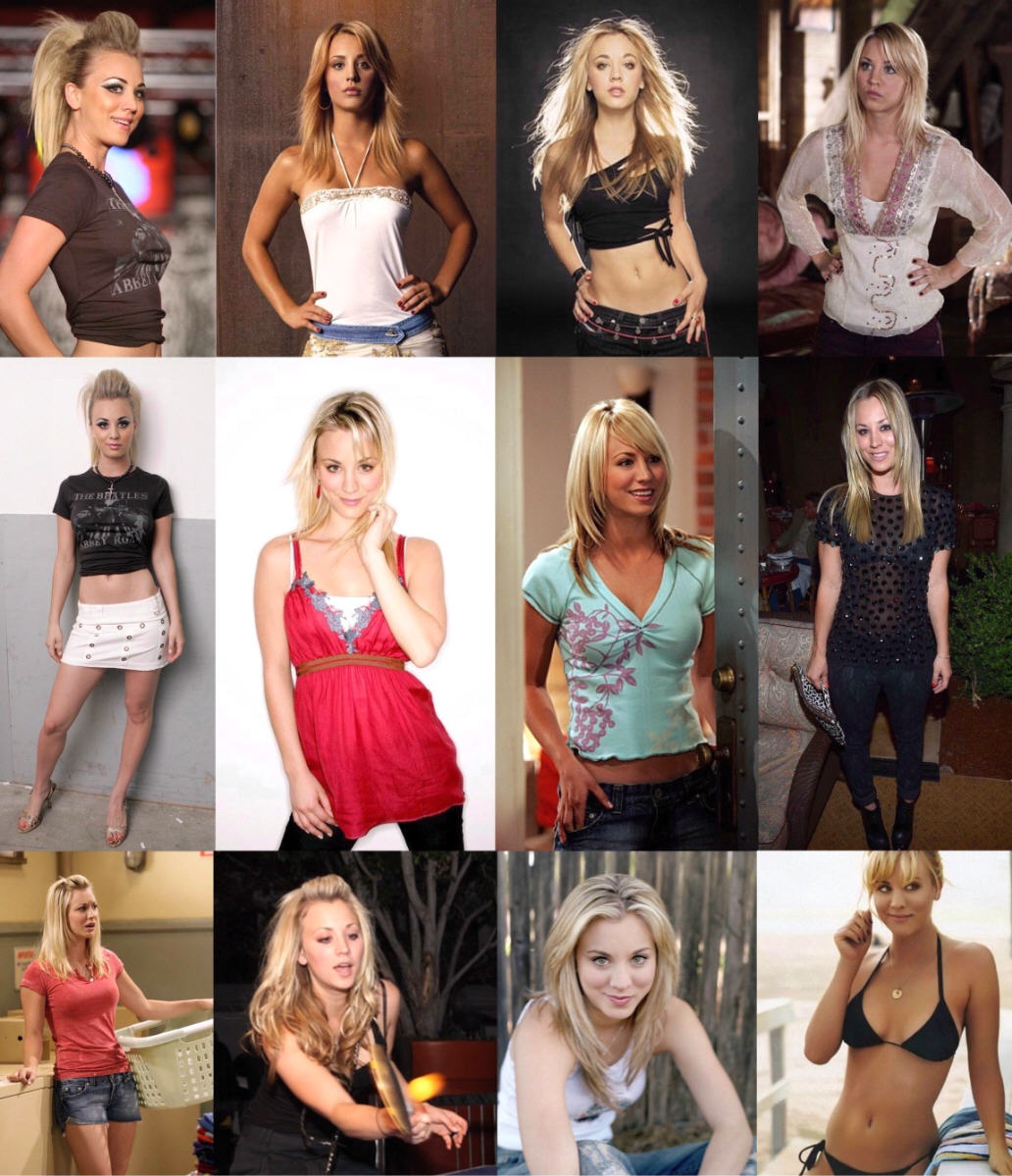This image collage features 12 portrait-mode photographs of Big Bang co-star Katy Coco, showcasing a range of outfits and poses. The collage is structured with images at the center being taller. 

In the top row, from left to right:
1. Katy sports a ponytail and a black shirt.
2. She wears a white shirt, with her arms on her hips.
3. Exhibiting a sexier look, she wears a midriff-baring top.
4. She dons another white-styled shirt, her hands placed on her sides.

In the second row:
1. Katy is dressed in a black crop top and a short white skirt, with her arms by her sides.
2. She wears a red dress paired with a white undershirt, her left arm under her chin and her right arm hanging down.
3. In a light blue shirt, her arms are at her sides.
4. She is seen in black jeans and a black shirt, with her arms down.

In the third row:
1. Katy is in a pinkish shirt and jean shorts, her left arm extended out and her right arm down.
2. She sports a black shirt and jeans, her arms outstretched.
3. Wearing a white shirt, her arms outstretched, she gazes at the camera.
4. In a black bathing suit, she displays her torso with her right arm up by her eyes and her left arm hanging down.

The images vary in style, featuring professional photo shoots, candid snapshots, potential screen captures from performances, and even a possible runway photograph, collectively capturing Katy Coco in diverse poses and settings.